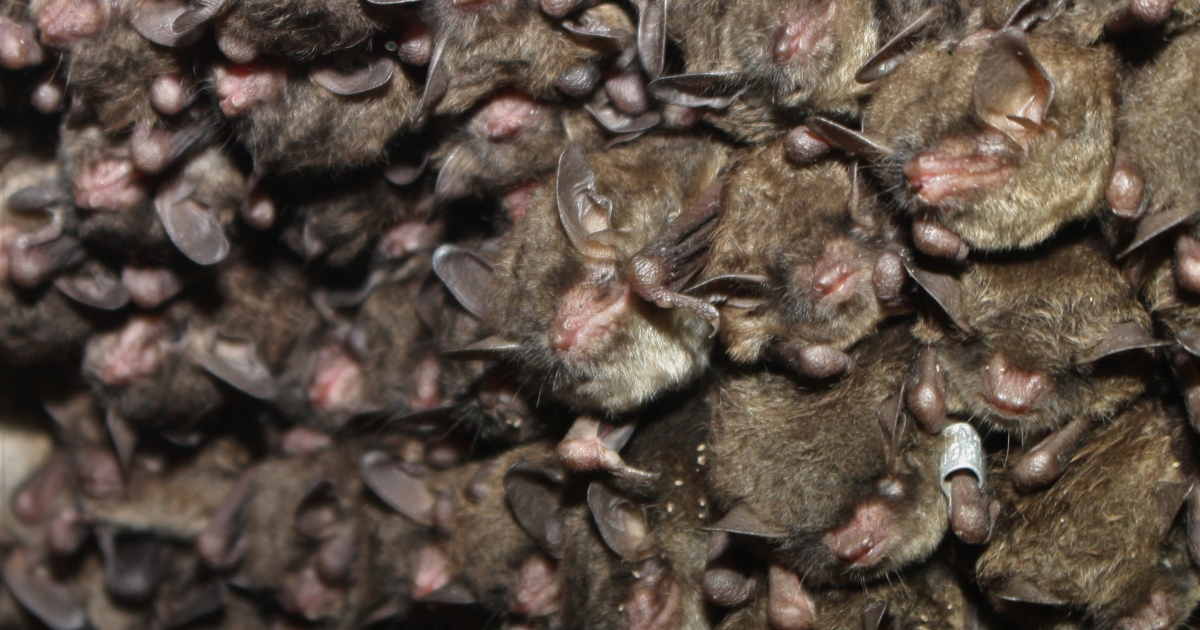The image depicts an indoor setting densely populated with bats clinging to the ceiling. The bats have brown fur, with some appearing light brown and others dark brown. Their wide mouths are notably red, and they feature long ears. The image shows an array of shapes and colors, including light brown, light pink, and light white, creating an abstract visual. The right half of the photograph is clear, providing detailed views of the bats, while the left half is fuzzy and less discernible. As a rectangle-shaped image, there are no borders, and the bats appear crumpled against each other, covering the surface without any spaces in between.